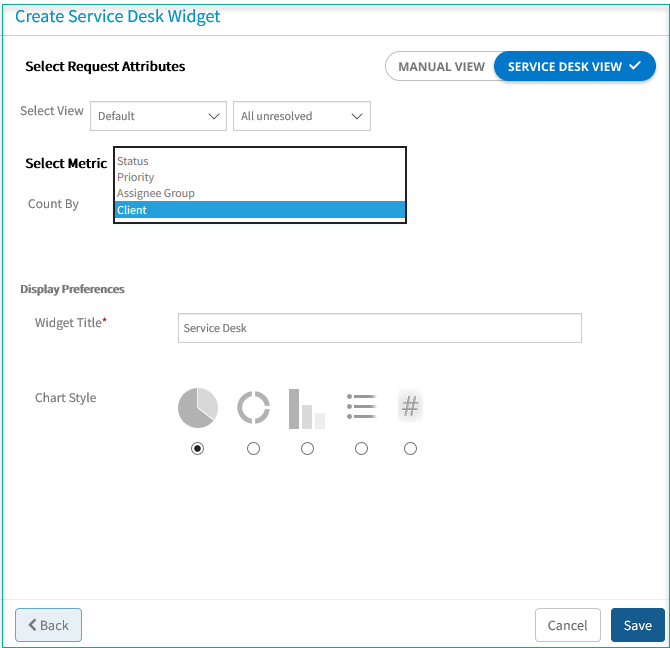This is a screenshot capturing a dialog box from the tool called "Create Service Desk Widget." The pop-up window has a clean and straightforward design, featuring a white background with a thin green outline framing the entire box. At the top, a simple blue header reads "Create Service Desk Widget." Just below the header, a horizontal gray line serves as a divider.

The main section begins with a bold black heading: "Select Request Attributes." Adjacent to this heading, there is a toggle menu that allows switching between "Manual View" and "Service Desk View." The current selection is "Service Desk View," highlighted in blue with an accompanying check mark indicating that it is active.

Below the toggle menu, there are two dropdown boxes labeled "Select View," showing options "Default" and "All Unresolved." Farther down, an option named "Select Metric" is visible, offering several choices: Status, Priority, Assigning Group, and Client. The open "Select Metric" box partially obscures another option titled "Count By."

Further below, there is "Display Preferences" followed by "Widget Title," which has a text box pre-filled with the word "Service Desk." The final section is labeled "Chart Style," presenting five different chart style options, with the current selection being a pie chart.

This dialog box is intended to help users customize and create service desk widgets, allowing them to select specific attributes, views, and visual display preferences.